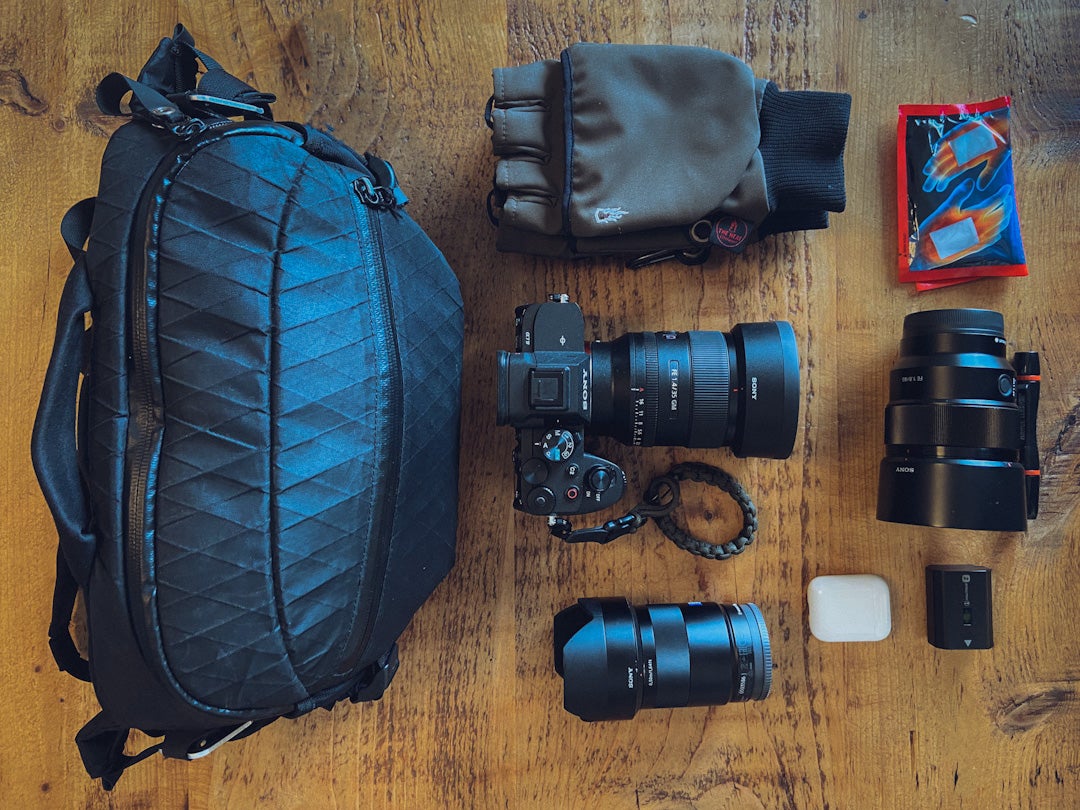The overhead photo showcases a collection of photography gear laid out on an orange-brown wooden table. On the left side, there's a dark blue camera bag with a strap and visible zippers. Resting on top of the bag are a pair of fingerless gloves, featuring a mitten cover and ribbed wrist cuffs, which are primarily black with grayish tones. To the right of the gloves, there's a red and blue package displaying a drawing of hands, possibly hand warmers. The central focus is a camera pointing to the right, equipped with a large lens and an attached wrist strap. Surrounding the camera are various camera lenses, one of which is stationed directly beneath it. Above the lenses lies a pair of Apple AirPods, adding to the assortment of equipment on display. All items are meticulously arranged on the wooden platform, highlighting their organized setup.